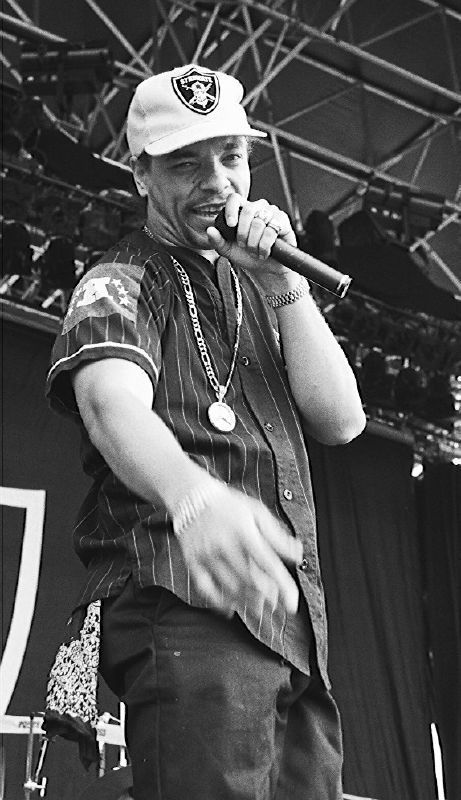In this black and white photograph, a Hispanic man is performing energetically, likely rapping into a microphone held close to his mouth with his left hand. He is adorned with a distinctive, large gold disc necklace that rests prominently on his chest. His outfit features a collared, button-down shirt with vertical stripes, paired with black pants. Additionally, he sports a white Raiders ball cap and a wristwatch with an expandable band on his left wrist. Positioned on a stage in front of a backdrop of black curtains, the man appears to be engaging directly with his audience, possibly pointing and singing to someone in the crowd.